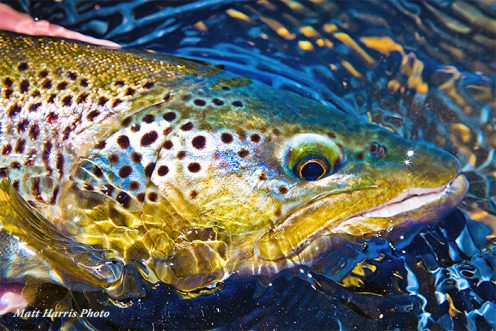This close-up photograph captures a striking fish, half submerged in a cyan and dark blue pool of rippling water. The fish's body is a mesmerizing mosaic of metallic gold, silver, and yellowish-green scales, interspersed with brown and black polka dots of varying sizes, creating a non-uniform pattern. The scales on its back sparkle prominently, emphasizing its otherworldly iridescence. Its large eye, encased for protection, is set deep within a pronounced socket and features a striking brown color with a black pupil, enclosed by a golden rim. This eye, along with the fish's vibrant scales, lends an almost regal appearance to the creature. The fish's coloration transitions beautifully from a bluish-green head to a yellow-gold hue around the gills and mouth, accentuating its natural elegance. The photographer's credit, "Matt Harris photo," is subtly inscribed near the bottom left corner, adding a professional touch to the pristine image.